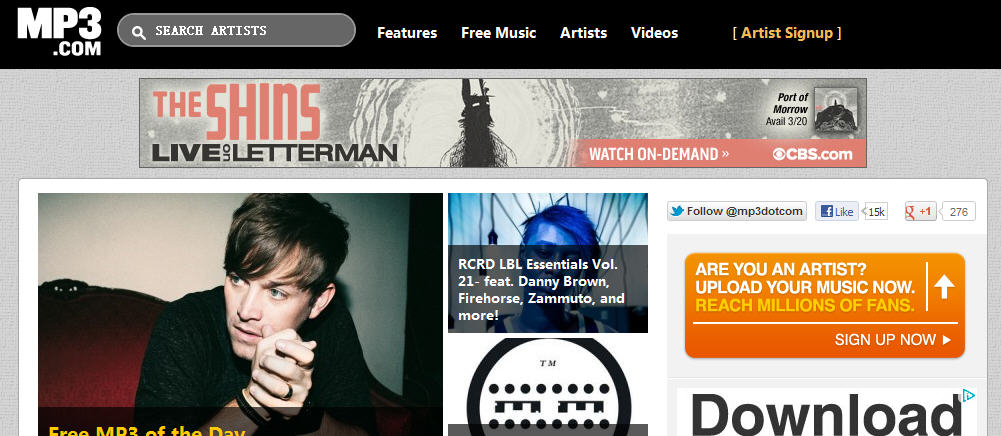This image, sourced from mp3.com, features a comprehensive layout showcasing various elements. In the upper left corner, the logo "mp3.com" is prominently displayed, with "dot-com" written in a smaller font beneath the "mp3". This section is framed by a black bar that spans the width of the image, creating a contrasting header. Adjacent to the logo on the right, there is a search bar labeled "Search artists". 

Below this header is a horizontal menu that includes the options: Features, Free Music, Artists, Videos. Further down, there's an invitation for users to sign up.

The background of the image is predominantly gray, but it is interrupted in the center by a striking banner. This banner, center-justified, reads "The Shins Live on Letterman" with a prompt below it to "Watch on Demand" via CBS.com. 

Dominating the lower portion of the image is a large white box. On the left side of this box, an individual is depicted sitting and facing the left. Overlaid on this section, the text "Free MP3 of the Day" is displayed. To the right of this person, the word "Download" is visible, accompanied by a call-to-action box that says, "Are you an artist? Upload your music now."